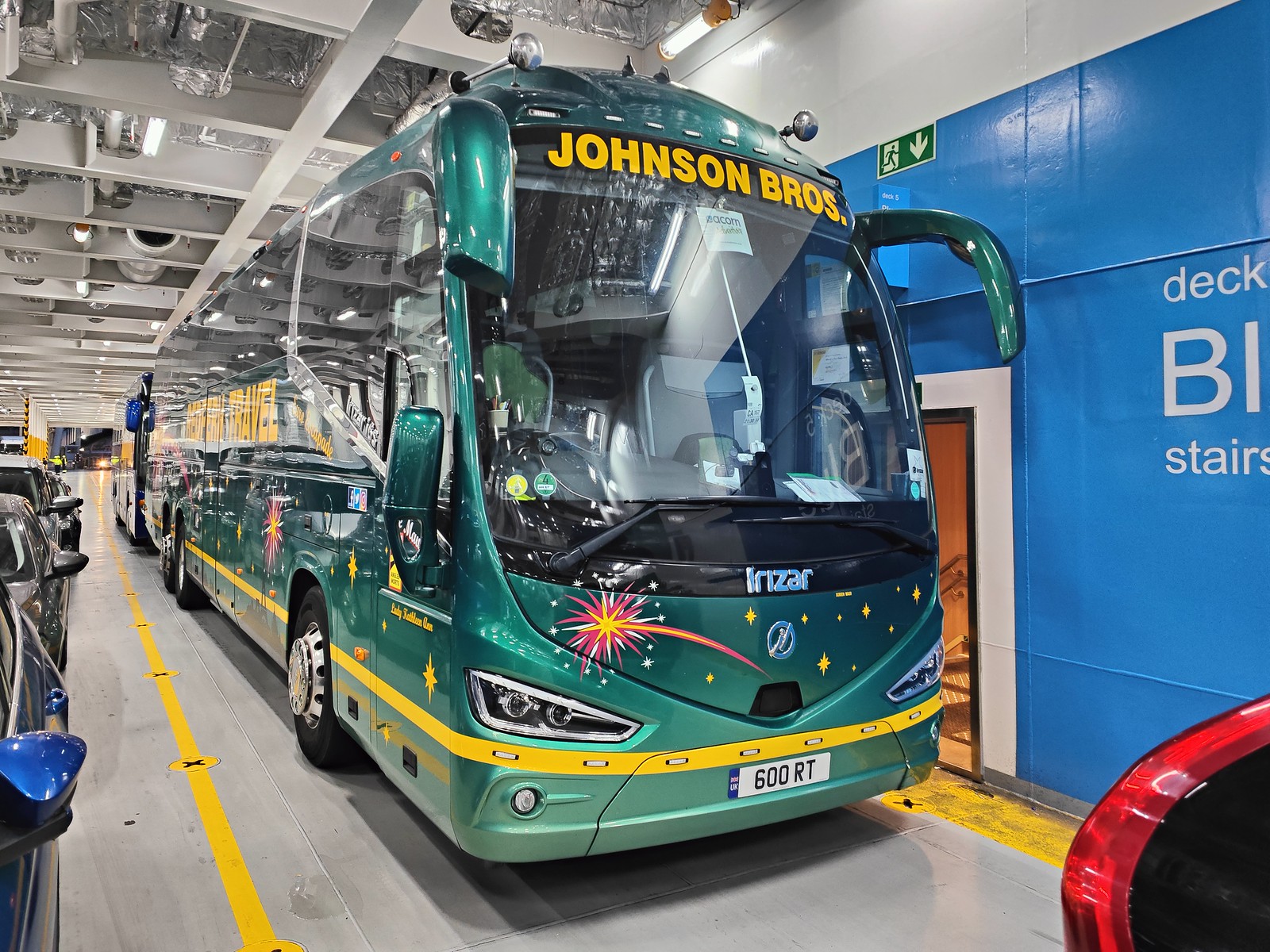The photograph showcases a large, aquamarine bus with colorful decorative elements, centrally positioned within an indoor facility that resembles a garage or depot. The bus, identified as an Inzar model, features an elaborate design with fireworks and shooting stars in pink, yellow, and green hues adorning its front and sides. Its prominent windshield displays the name "Johnson Bros" in bold yellow print. The vehicle, which has black wheels with silver hubcaps, is partially obscured by a glare on the windows, reflecting the well-lit interior of its surroundings.

The facility's white ceiling is composed of rafters and beams intersected by metallic silver ductwork. The cement-like floor beneath the bus is marked with yellow lines. The bus seems to be positioned for either storage or maintenance, indicated by its inactive lights and stationary placement. To the left, cropped views of several cars, including a blue one showing just its side mirror, frame the bus, while behind it to the right, a bright blue and white wall features partial white text and a doorway trimmed in black. This door might serve for offloading passengers or access to other areas of the depot.